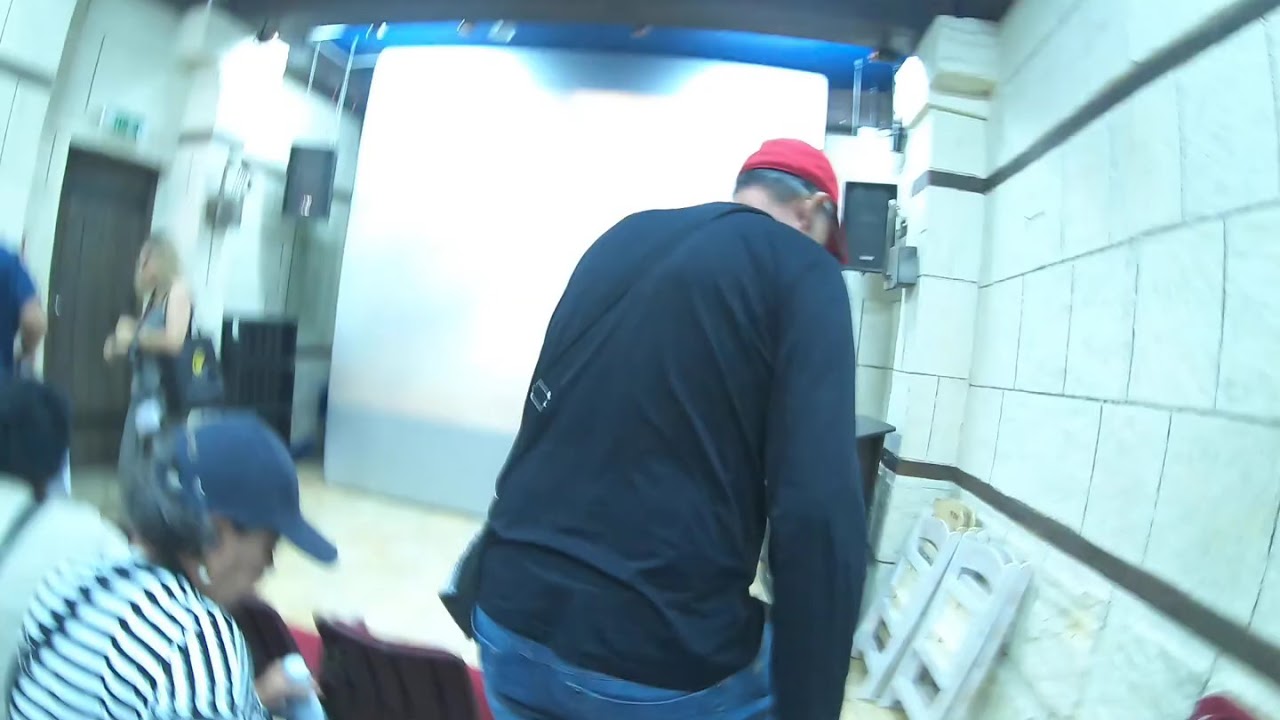The image shows a white-walled room with two speakers and a projector mounted on the ceiling. In the foreground, a man wearing a long-sleeved black shirt, a red hat, and blue jeans is prominently walking past, facing away from the camera. To the left, a woman with a blue baseball cap and a black-and-white striped shirt is seated and looking down, though the image is slightly blurry, making her hard to fully discern. In the background, there is a standing woman wearing a gray tank top, also seen glancing downward. The room also includes a door that is brown, white-tiled walls with black lines, and a white rubber floor. Overall, the scene captures a slightly blurry, bustling indoor environment.